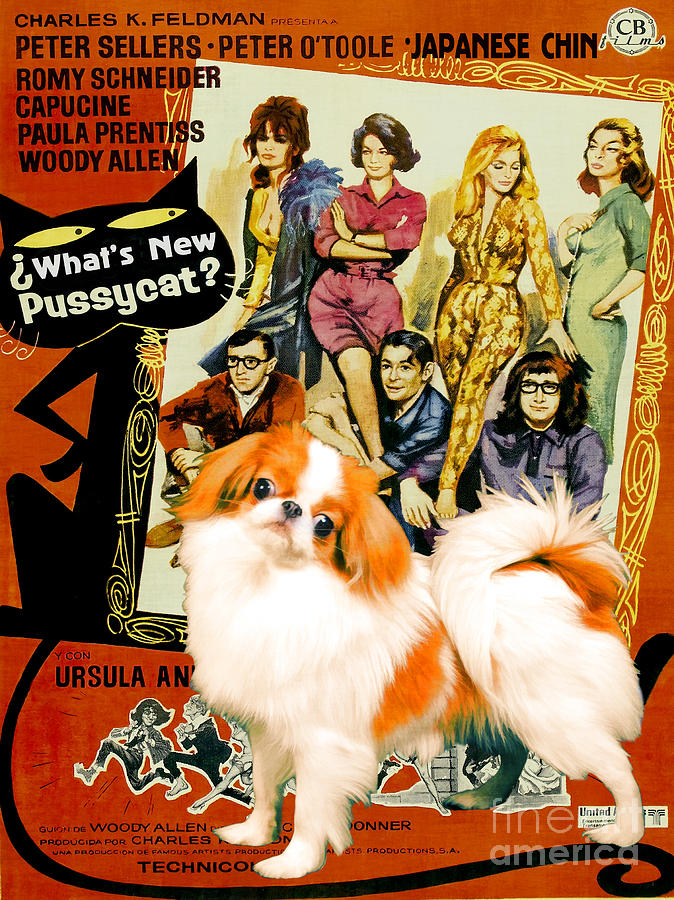The image represents a modern collage styled as a vintage movie poster or magazine cover. Dominated by an orange background, it prominently features text at the top that reads "Charles K. Feldman Presents: Peter Sellers, Peter O'Toole, Japanese Chin, Romy Schneider, Capucine, Paula Prentiss, and Woody Allen." The main illustration showcases an animated caricature of these stars. The scene is split into two tiers: the top displaying four women dressed in vibrant 70s fashion, and the bottom showing three men, including Woody Allen with his signature glasses, seated among the women. 

A notable feature is the black cartoon cat in silhouette with yellow eyes, labeled "What's New Pussycat?" Additional elements include a CB Films emblem in the top right corner and a Technicolor mention at the bottom. Superimposed upfront is a white dog with orange fur on its ears, sides, belly, and tail. The dog, seemingly incongruous with the vintage theme, hints at a modern collage approach. Scattered throughout the image are snippets of text mostly obscured by the dog's positioning, adding to the layered, chaotic aesthetic typical of a magazine cover bursting with information.

Overall, the poster combines retro cinematic elements with contemporary digital art, characterized by its vivid color palette of blues, yellows, reds, oranges, purples, and greens. The juxtaposition of classic and modern, highlighted by the oddly-placed dog, sets a playful tone reminiscent of 1970s pop culture.